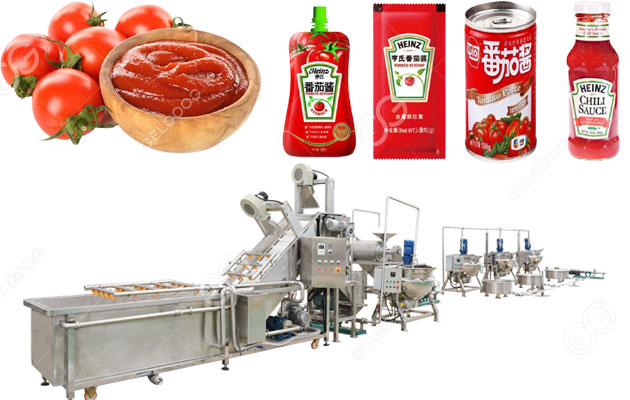The image is a detailed product photograph showcasing various Heinz-branded tomato-based products set against a white background. On the top left, a wooden bowl filled with ketchup sits adjacent to five plump, red tomatoes each with green stems. Moving towards the right, a lineup of four distinctive Heinz products is displayed: a squeeze bottle of tomato puree with Asian characters on its label, a metallic packet expected to contain ketchup, a can labeled "tomato paste" with a red label, and a glass jar of Heinz chili sauce. Below these products, occupying the bottom portion of the image, is a large, industrial machine designed for canning and packaging. This robust machinery features numerous interconnected components and control panels with green and red buttons, indicating its purpose in mass production for retail distribution. The image effectively ties together the end products with the industrial equipment used in their creation, hinting at the scale and sophistication involved in manufacturing these household staples.